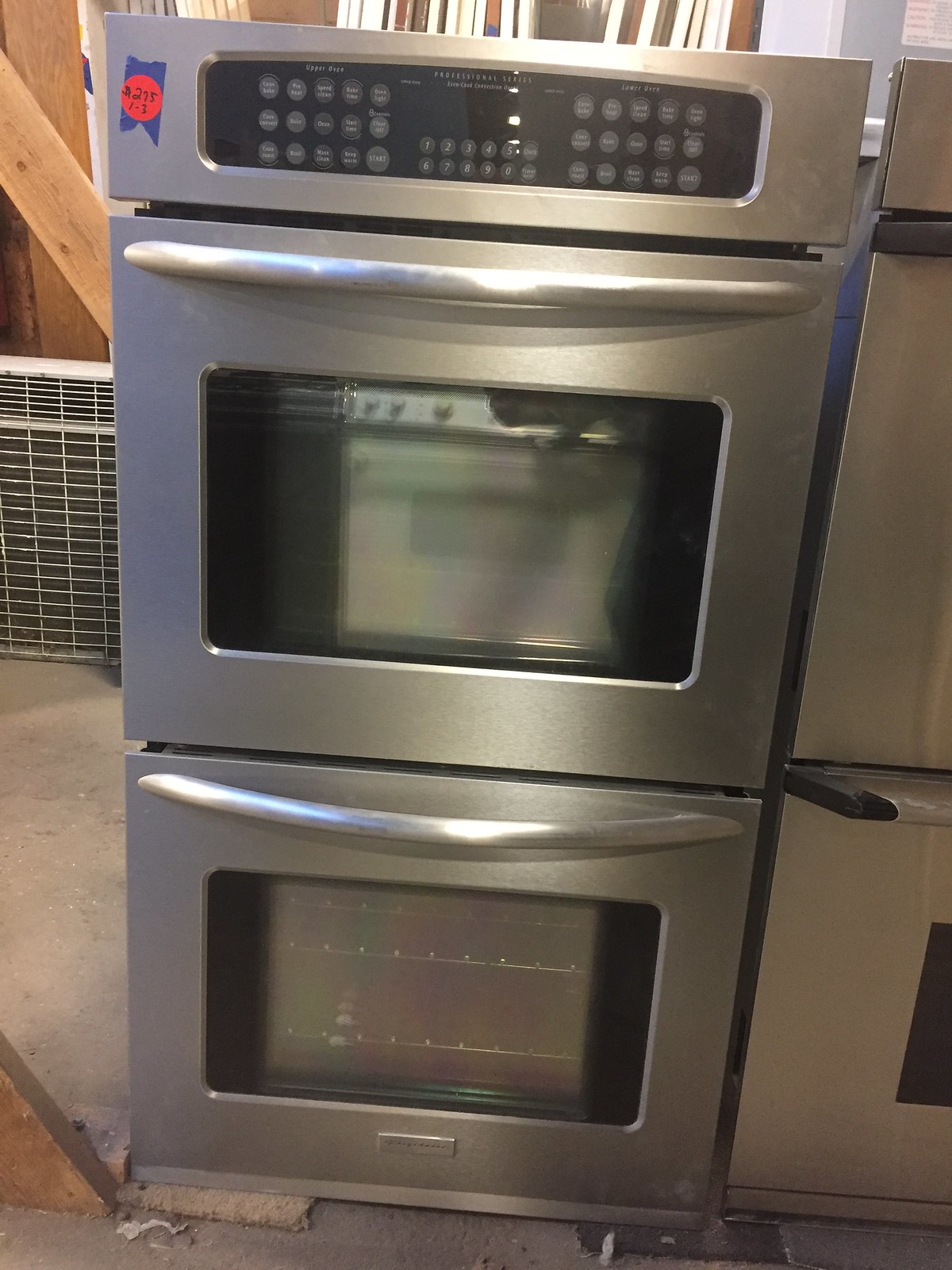The photograph captures a stainless steel double-decker oven, positioned on what appears to be a protective mat or carpet, potentially in a basement, garage, or storage area. The oven features a sleek design with black control pads at the top, accented by a multitude of flat buttons. The top oven door has a reflective glass panel, while the bottom door's glass reveals two metal racks inside. A blue sticker with a red circle is affixed to the left side of the control panel, though the text is indecipherable. The oven has chrome-like handles on both doors, which are arranged horizontally. The setting includes a cement floor and wooden panels in the background, with a sliver of another stainless steel appliance visible to the right. Additionally, a staircase, possibly made of wood, is faintly seen on the left side of the image, contributing to a sense that the ovens are awaiting installation.